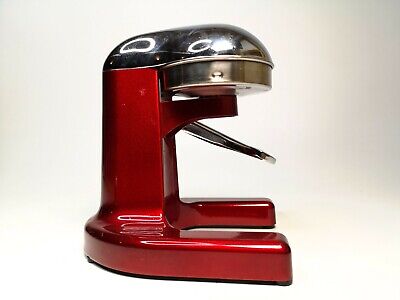The image presents a detailed, realistic depiction of a red household appliance that closely resembles a stand mixer but with some unfamiliar features. The appliance, likely positioned in a modern kitchen, has a sleek design combining a bright, shiny red base with a highly stylized chrome top. Notably, an arm extends from the red base towards the silver top, featuring a conspicuous silver protrusion that adds to the intrigue of the appliance's function. The bottom of the appliance has a distinctive horseshoe shape, providing stability and aesthetic appeal. While its exact purpose remains ambiguous, suggestions range from it being a can opener or a soda opener to perhaps even a piece of cutting-edge technology or a milkshake maker. The unique design and the mysterious proboscis-like feature make it a captivating subject of curiosity.